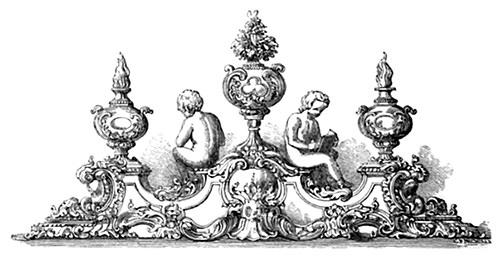The image showcases an intricate black and white illustration with a strong influence of classical and biblical iconography. Central to the artwork are two cherubic young men, positioned nude on an angular, concrete-like wall adorned with ornate embellishments that resemble an old European style. The wall features curving, arched designs and scroll-like patterns interspersed with vines extending across its surface. At the heart of the composition, a large, circular statue, possibly an urn or vase, stands prominently, topped with a flourishing bouquet of flowers or small foliage. Flanking this central statue are two smaller, similarly designed pedestals, each supporting additional urns with elaborate decorations. The cherub on the right is engaged in reading a book, while the one on the left has his back turned, obscuring his activity. The elevated platform they sit on casts subtle shadows, adding depth to the illustration. The detailed embellishments and the figures’ serene postures evoke a timeless, classical ambiance that enhances the scene's overall decorative and artistic appeal.